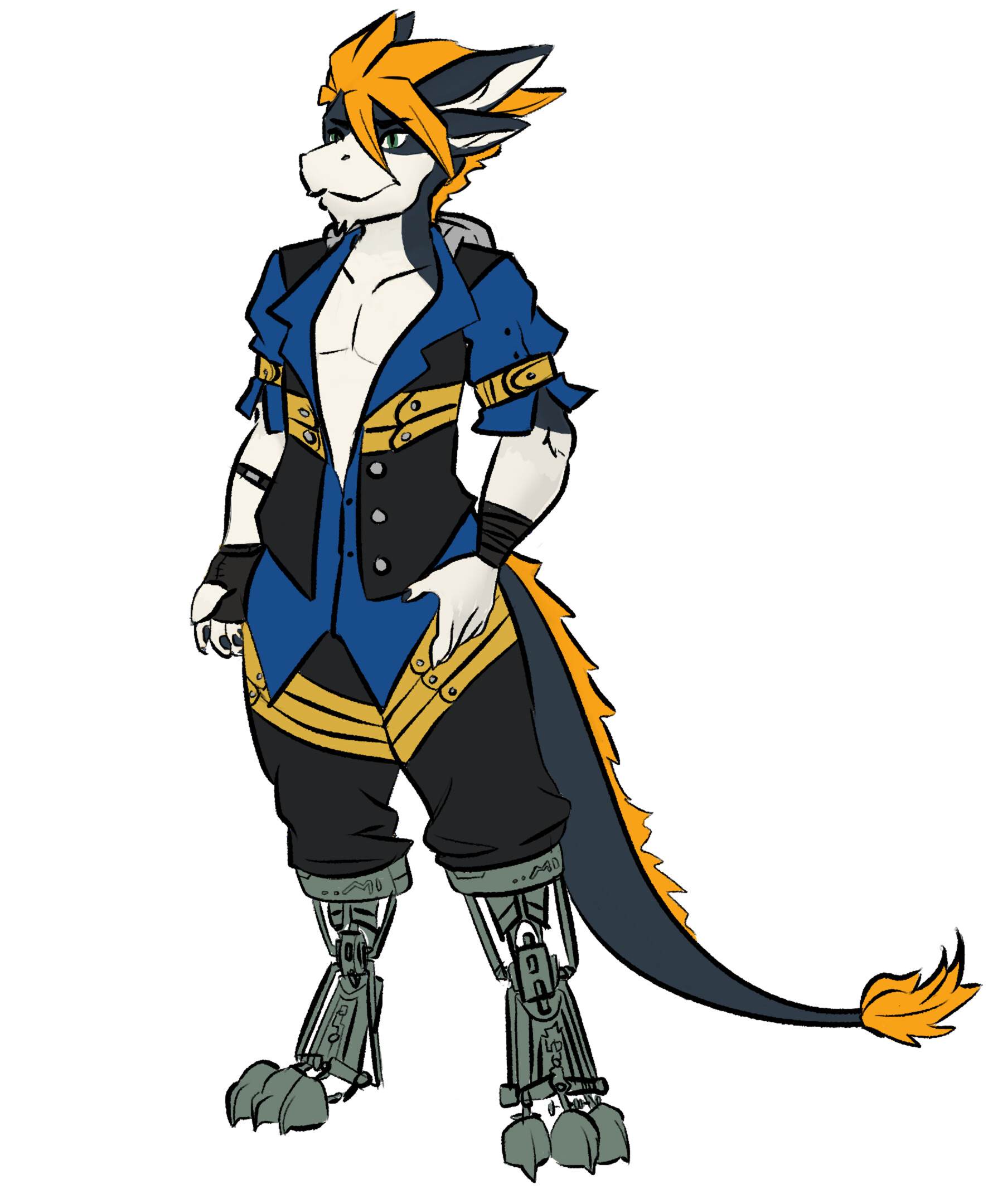The image portrays a detailed cartoon figure with a combination of human, animal, and robotic features. The character has a distinctive head reminiscent of a donkey with large, clear, and long ears and an orange, fluffy mane. Its upper body displays a humanoid form, with the chest exposed beneath an unbuttoned, predominantly navy blue and black vest adorned with gold accents and formal points on the sleeves.

The figure's attire consists of black pants with gold stripes, and it flaunts a black tail featuring orange highlights and spikes, which resembles that of a lion or dragon. Notably, the legs and feet of the character are mechanical and clawed, showcasing metal ankles and feet, adding to the character's unique blend of organic and mechanical elements. The overall appearance is clean, with some wristbands as additional details, and the figure exudes a certain anime-like charm with its unique smile and expressive look.